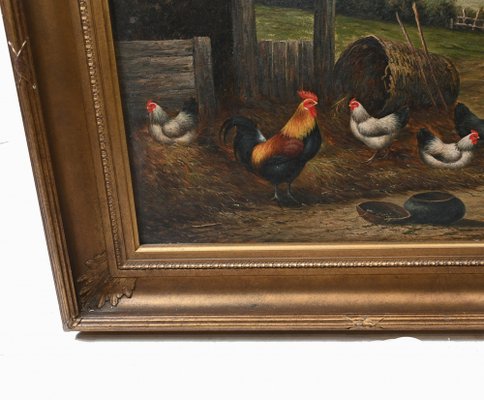This image shows the bottom left corner of a framed painting, highlighting a rural scene with chickens. The ornate, dark brown wooden frame encloses a depiction of four chickens on a straw-covered ground. The main focus is a black rooster with a tan head, red eyes, and the characteristic red comb and wattle. Surrounding it are three white hens with black detailing. One hen is walking, while the others are either resting on the straw or positioned around the rooster. Behind the chickens, there’s a tipped-over barrel, a gray pot with a lid slightly ajar, and some wooden fencing that encircles the scene. The backdrop bursts with earthy tones, predominantly shades of brown, accentuated by the rustic hay and wooden elements.